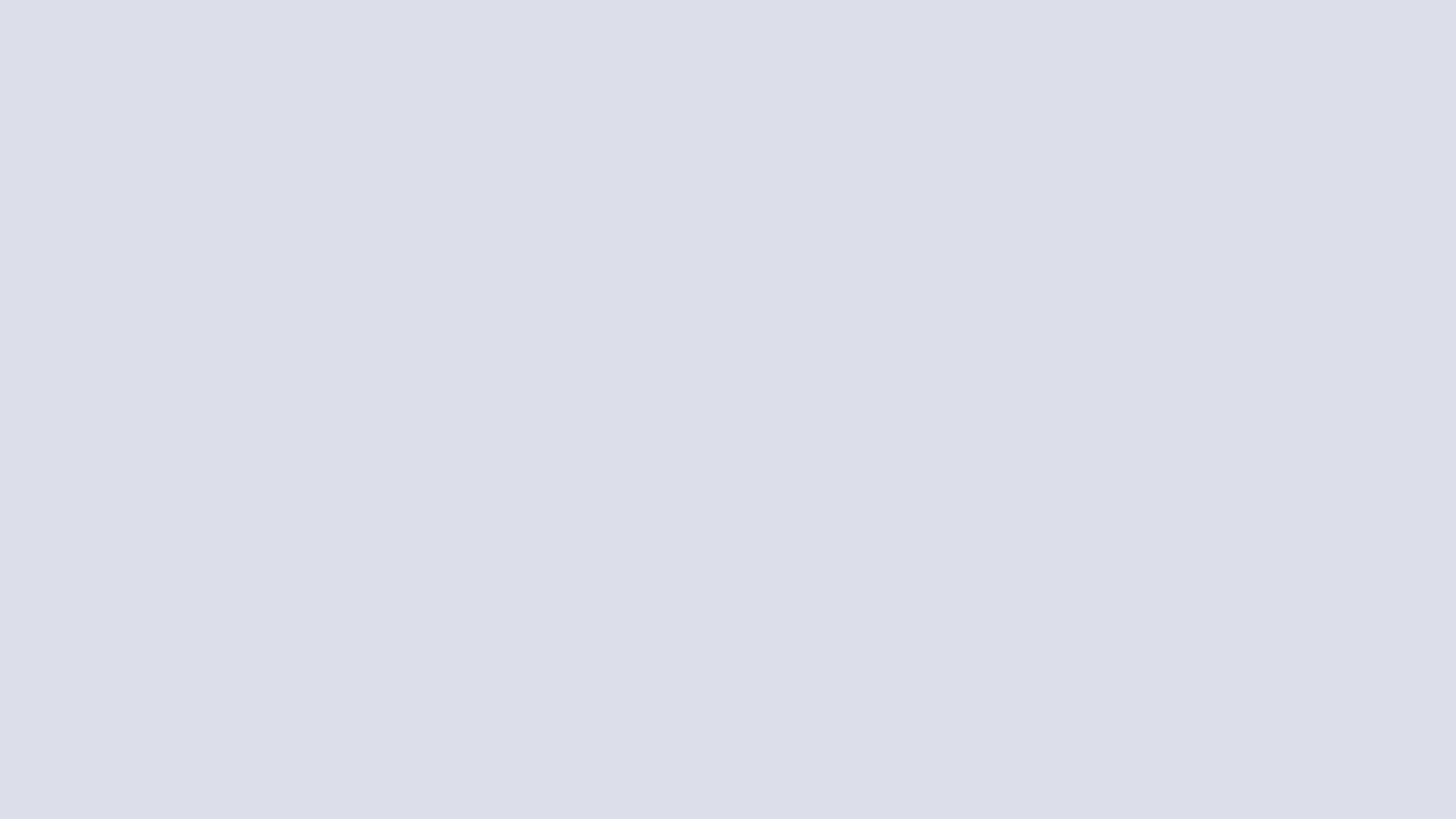A simple, unadorned image features a medium-gray rectangular box set against a pristine white background. The gray box, uniform in color without any shading or texture variations, extends longer horizontally than it does vertically, suggesting an intentional rectangular shape. There are no images, text, outlines, or labels within or around the box—its contents, if any were intended, are absent. The edges of the box seamlessly transition into the white surrounding it, devoid of any borders or markings. This minimalist composition could potentially be indicative of a placeholder or an error within a digital context where content was meant to appear but is conspicuously missing.